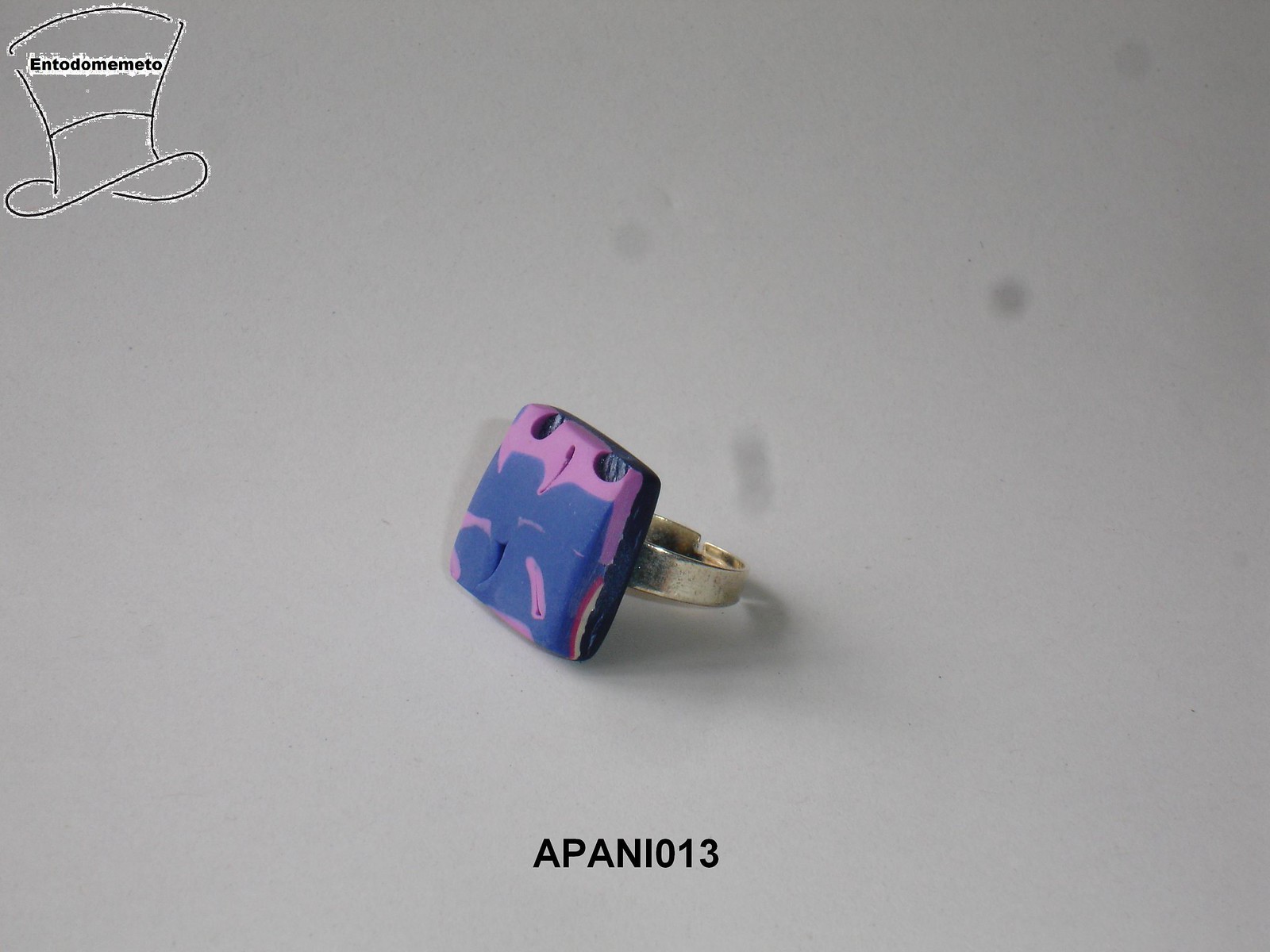The image depicts a gold ring set against a gray background. In the center of the image, the ring features a prominent, unusual square-shaped stone that appears to be made of plastic, rubber, or a similar material. The stone, approximately the size of a fingernail, showcases a vibrant mix of hot pink, dark blue, and hints of red and yellow on its top surface, while resting on a black base. Below this stone, the text "APANI 013" is visible in black letters. The background also has some smudging of blackish-gray colors, especially in the upper right corner, and a watermark on the upper left side featuring a top hat with the word "Entodomento" inscribed on it.